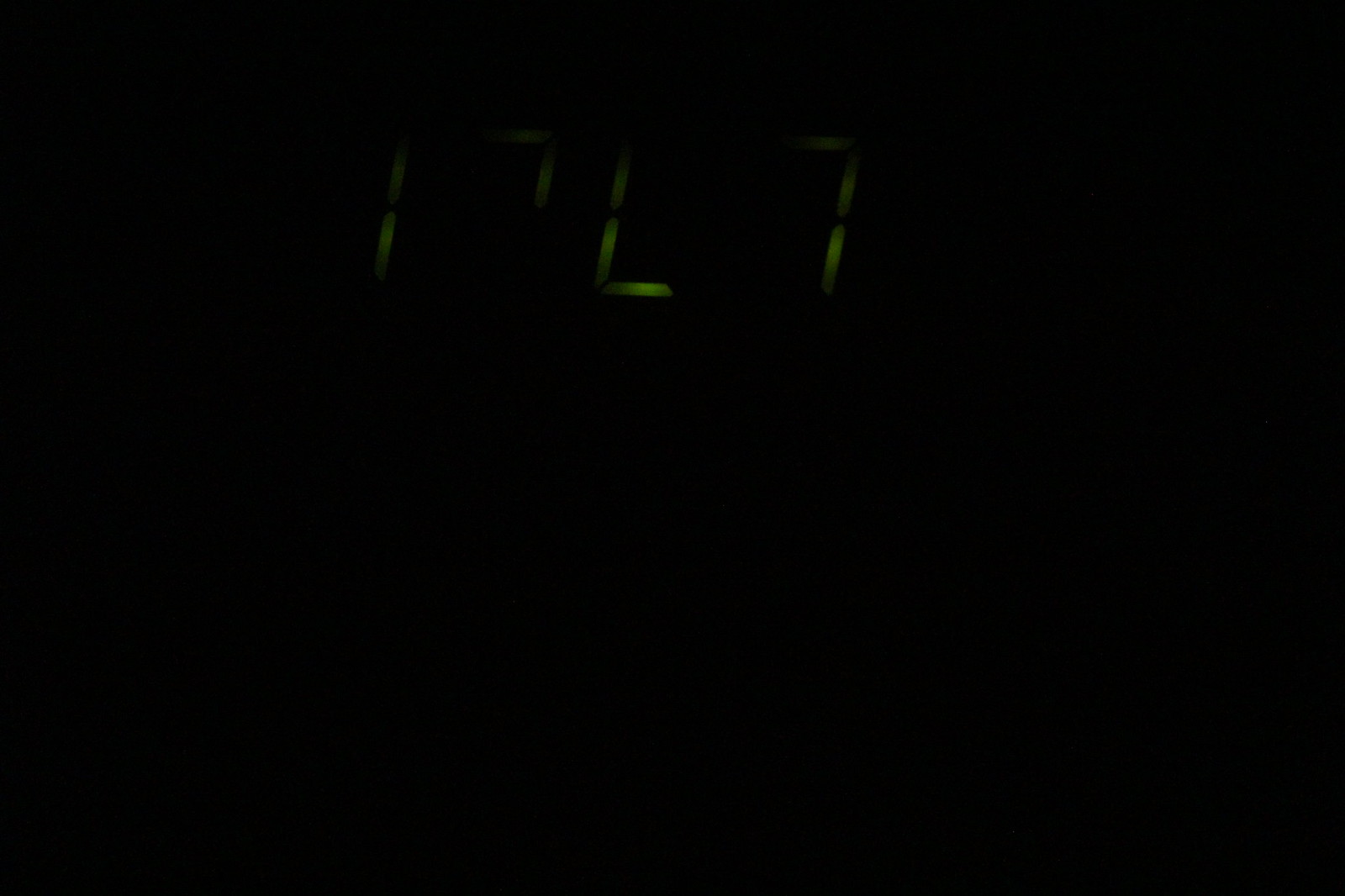The image is predominantly black, covering approximately 95% of the frame. A faint shade of green emerges from the top, suggesting remnants of a digital interface. The sparse green areas hint at what might have been numerals or letters, possibly parts of a digital clock. Specific details include small green sections resembling an "I" and an "L," as well as two vertically aligned green dots. The overall impression is of an old digital display, now almost entirely obscured by blackness, with just enough green to suggest its former functionality.